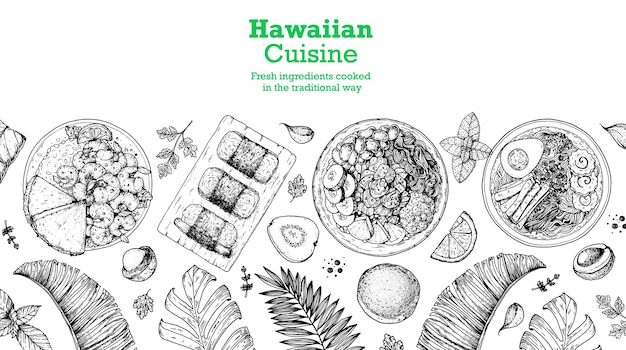Highlighted by green text that reads "Hawaiian cuisine, fresh ingredients cooked in the traditional way," this digitally-created advertisement showcases an array of foods through detailed black-and-white line drawings. At the bottom of the image are plates filled with various traditional Hawaiian dishes and decorative elements like monstera leaves and ferns. The depicted foods include fruits such as avocados, orange or lemon slices, and possibly pears or apples. Above the fruits, the image features actual meals: on the top right, there's a bowl of ramen with a soft-boiled egg, noodles, and vegetables. To the left of the ramen is a bowl containing assorted vegetables, and further left is a piece of spam musubi (rice with spam wrapped in seaweed). To the far left, a plate with breaded shrimp, rice, vegetables, and possibly pineapple is shown. Despite the monochrome palette, the intricate arrangement and detailing of the food items make the image both engaging and visually appealing, suitable for a restaurant advertisement or a business card.